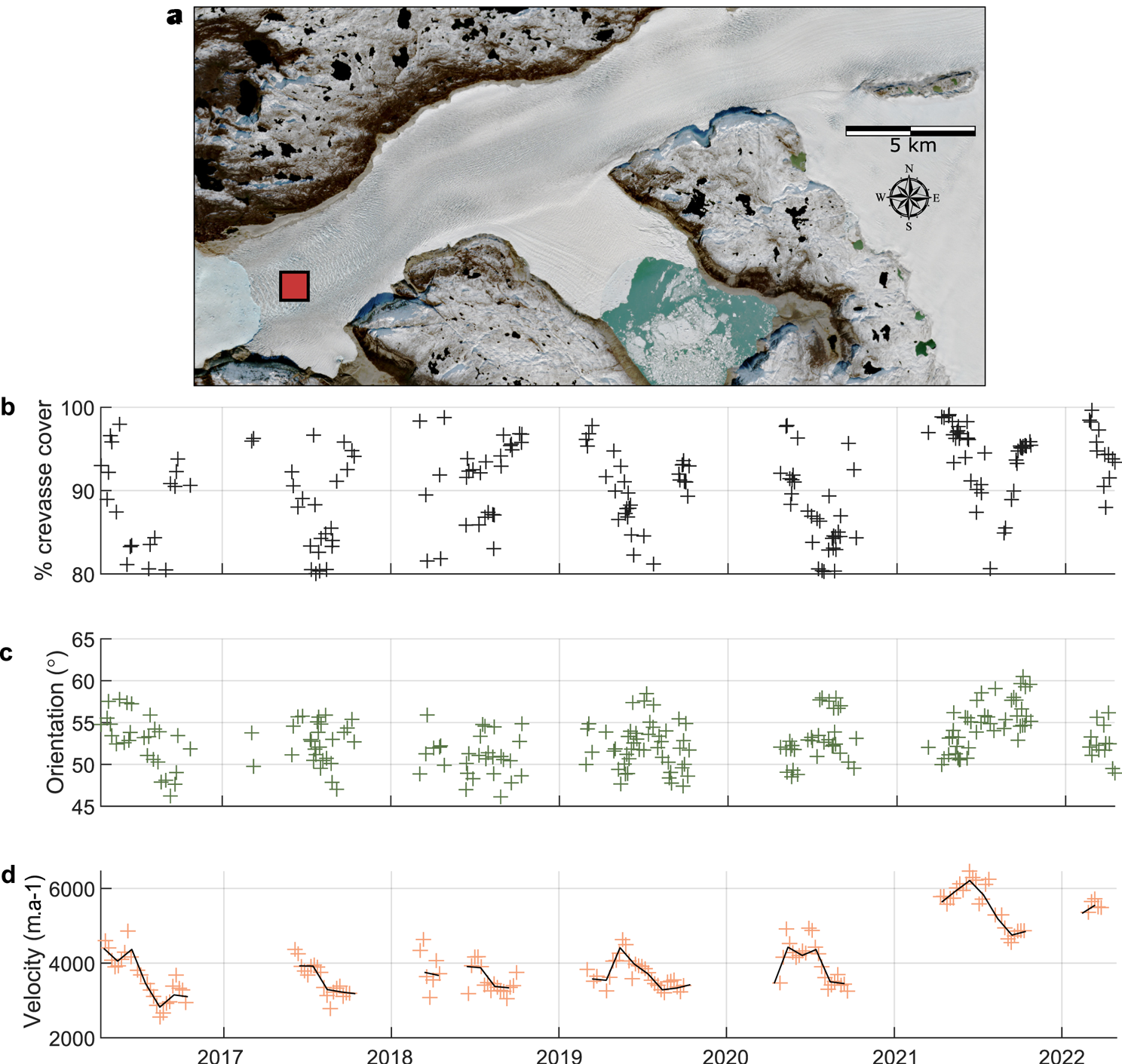The composite image consists of a scientifically detailed map and three illustrative charts. The top portion of the image, labeled A, displays an aerial or satellite photograph depicting a frosty landscape with two landmasses separated by a possibly frozen waterway or river. In the photo, a red square marks a specific location near the river's mouth. Positioned in the top-right corner is a northeast-southwest compass rose, and beside it, a scale bar indicating a distance of five kilometers spans about a tenth of the photo's width.

Beneath the photograph, three scatter charts labeled B, C, and D provide analytical data. 

- Chart B, titled "Percent Crevasse Cover," spans values from 80 to 100 and is populated with evenly distributed black plus signs. 
- Chart C, labeled "Orientation," ranges from 45 to 65 with green plus symbols scattered throughout. 
- Chart D, titled "Velocity (M·A⁻¹)," ranges from 2,000 to 6,000 and features data points connected by lines, indicating trends over time. The x-axis of chart D is marked with the years 2017 through 2022. 

Overall, this image is a visual and quantitative analysis of a geographical area, offering insights into crevasse cover, orientation, and velocity metrics over a five-year period.